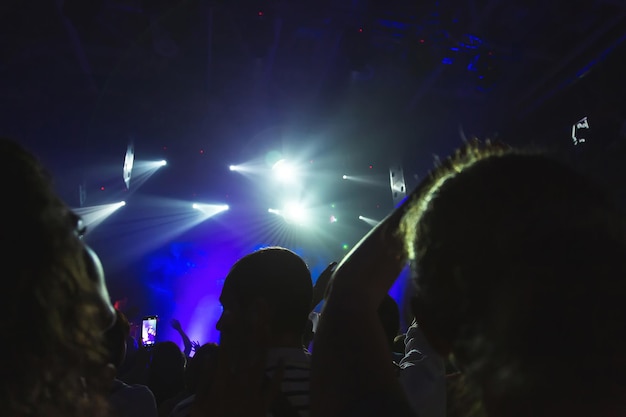The image captures the view from the back of a large, densely packed crowd at a concert, with many heads and raised arms visible. The scene is dimly lit, accentuated primarily by bright white stadium lights illuminating patches of the audience. The foreground displays a silhouetted man in the center, flanked by two indistinct heads to the left and right. A cell phone is held up to the left of the man's head, capturing the moment. The stage area, somewhat obscured, is bathed in blue and purple smoky effects, contributing to the concert atmosphere. The picture reflects the perspective of attendees positioned far from the stage, reminiscent of an experience where despite poor seating, the shared excitement of the concert pervades the ambiance.